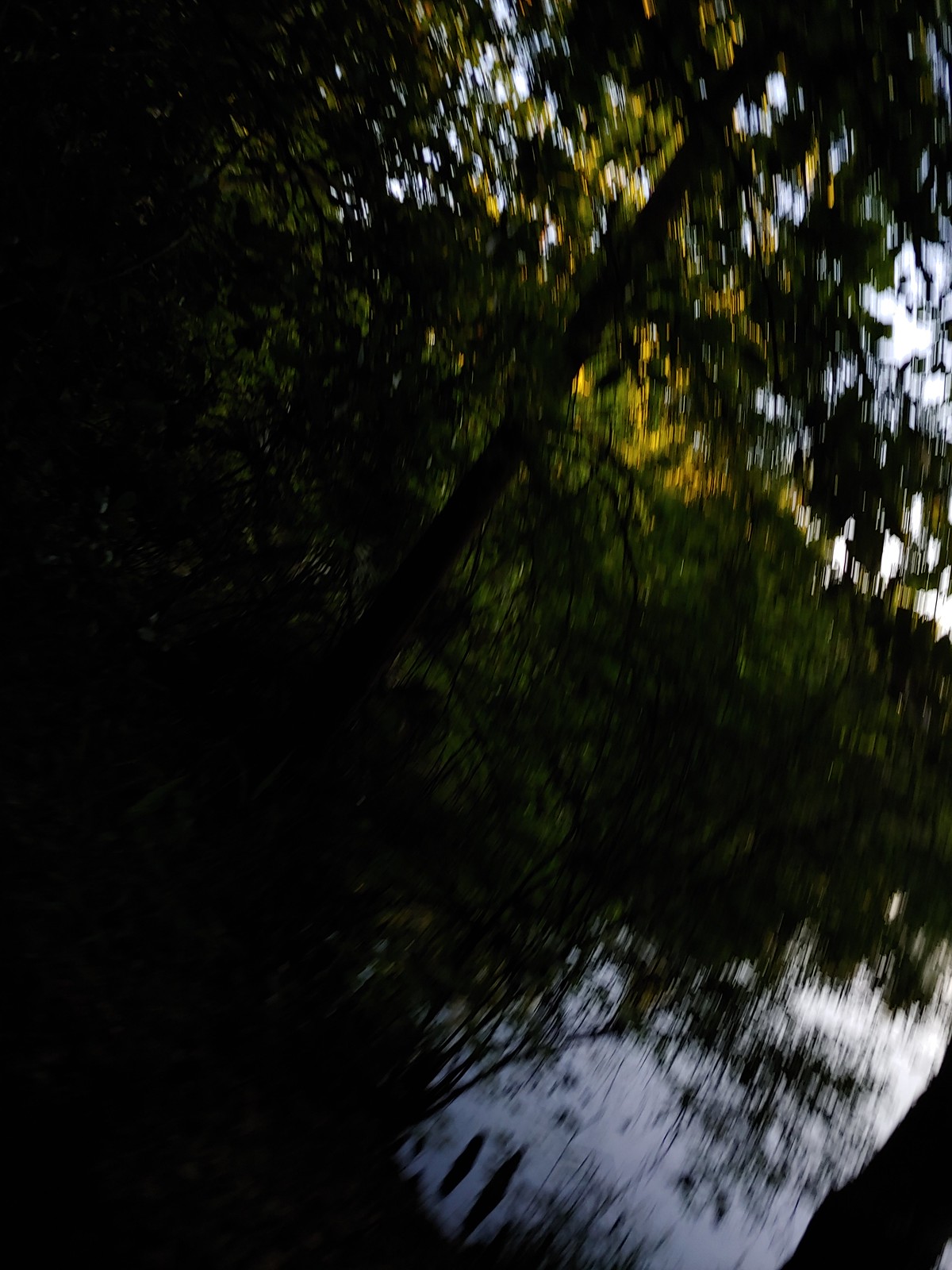The image is a blurry, color photograph in portrait orientation taken during the day. The frame is dominated by a dense canopy of trees, with foliage in varying shades of green and yellow, and very few gaps revealing an overexposed, bright sky. The lack of fine detail suggests it might have been taken accidentally or with an unsteady hand. The upper right corner of the image shows patches of sky with sunlight filtering through the leaves, while the lower right corner reveals what seems to be the surface of water, interspersed with grasses or bull reeds. The left side of the photograph is almost entirely in shadow, creating a stark contrast against the lighter areas. There are no people, animals, or buildings in the image, and the photograph lacks professional quality.